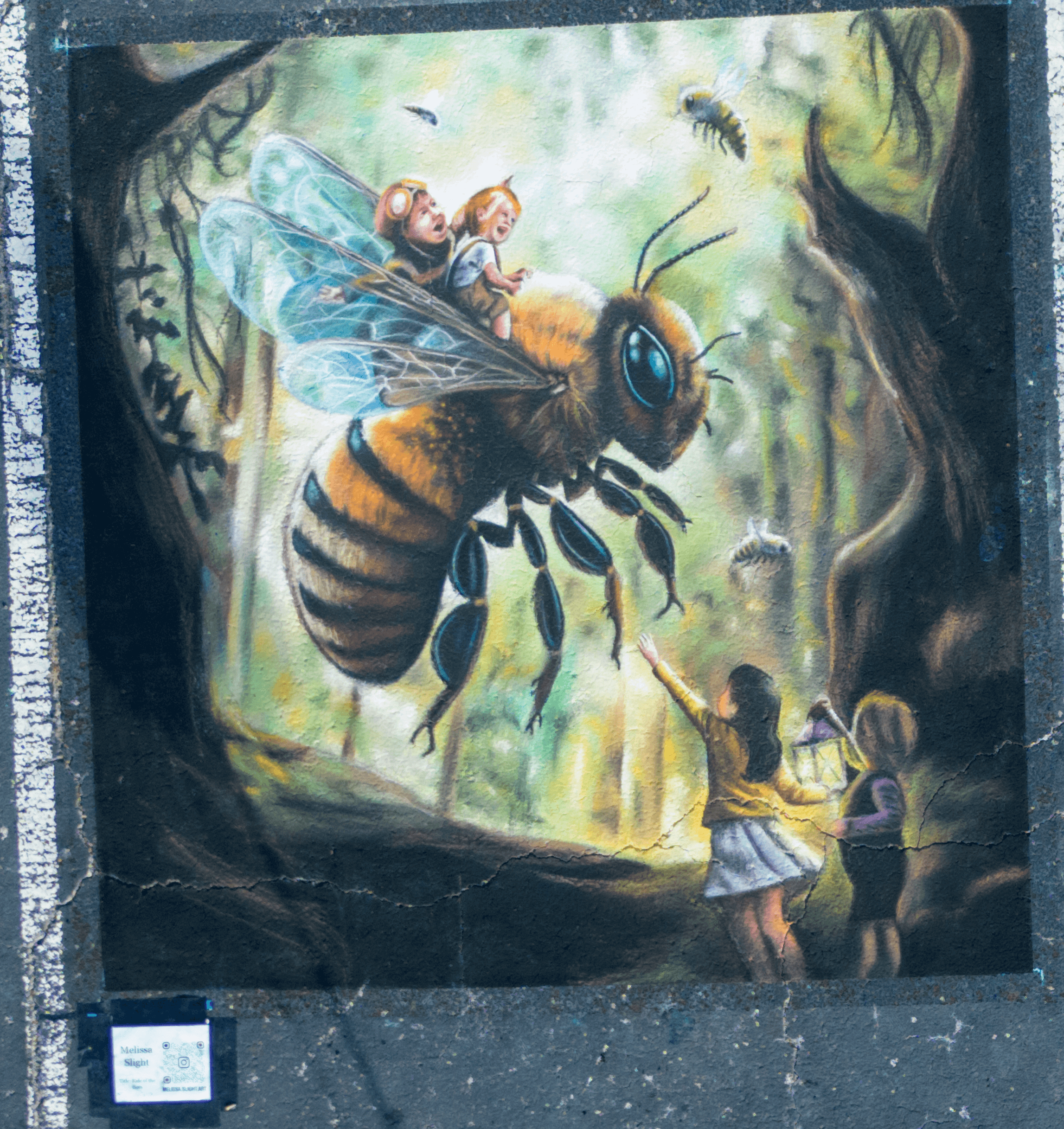This vertically rectangular illustration depicts a whimsical outdoor scene bathed in natural light, likely inspired by a children's fantasy story. The central focus is a gigantic bee facing rightward, with an older figure, possibly an adult wearing flying goggles, and a small child riding on its back just in front of its wings. Below, in the lower right corner, a miniature boy holding a lantern and a girl reaching up stand amidst a brown clearing. The background reveals a shadowy, mystical forest with more bees hovering in the distance and trees bordering both sides of the image. A blue border frames the scene, resembling the spine of a book. In the lower left corner, an unreadable white square adds a touch of mysterious text to the overall composition.